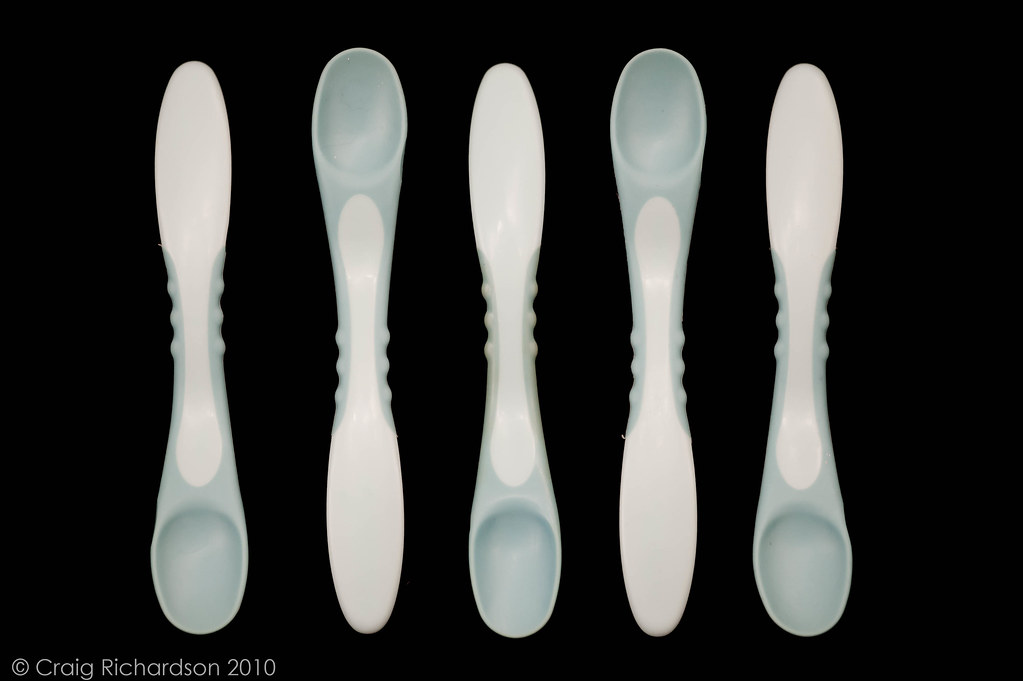This photograph depicts five baby spoons arranged on a solid black background with the copyright text "Craig Richardson 2010" in white letters in the bottom left corner. The spoons feature a pattern of alternating positions, with handles pointing up and down sequentially from left to right. The spoons have a light blue or sage green spoon area and white handles, which appear to be made of plastic. Each handle has three bumps along either side, designed for better grip, indicating that these are likely children's utensils. The alternating arrangement and the distinctive color pattern, where the spoon part features a hint of color blending into the white handle, create a visually engaging display.